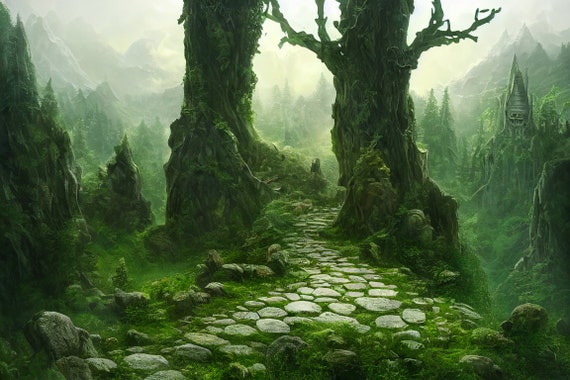The image depicts a green, foggy forest with a dark, eerie atmosphere, reminiscent of a horror show or dark fantasy setting. Central to the scene are two large, partially moss-covered tree stumps, flanking a winding cobblestone path where moss has grown through the stones. This path appears ancient, as if it has been trodden by people long ago, leading deeper into the misty, moss-laden woods. The forest background is shrouded in a white haze, concealing full details but revealing twisty, old trees and pointed hills or rock structures. Among these, on the right, is an indistinct object resembling a metal sphere, also moss-covered. The entire scene is cast in an airy green fog, with rock formations scattered throughout, enhancing the haunted feel of the forest.